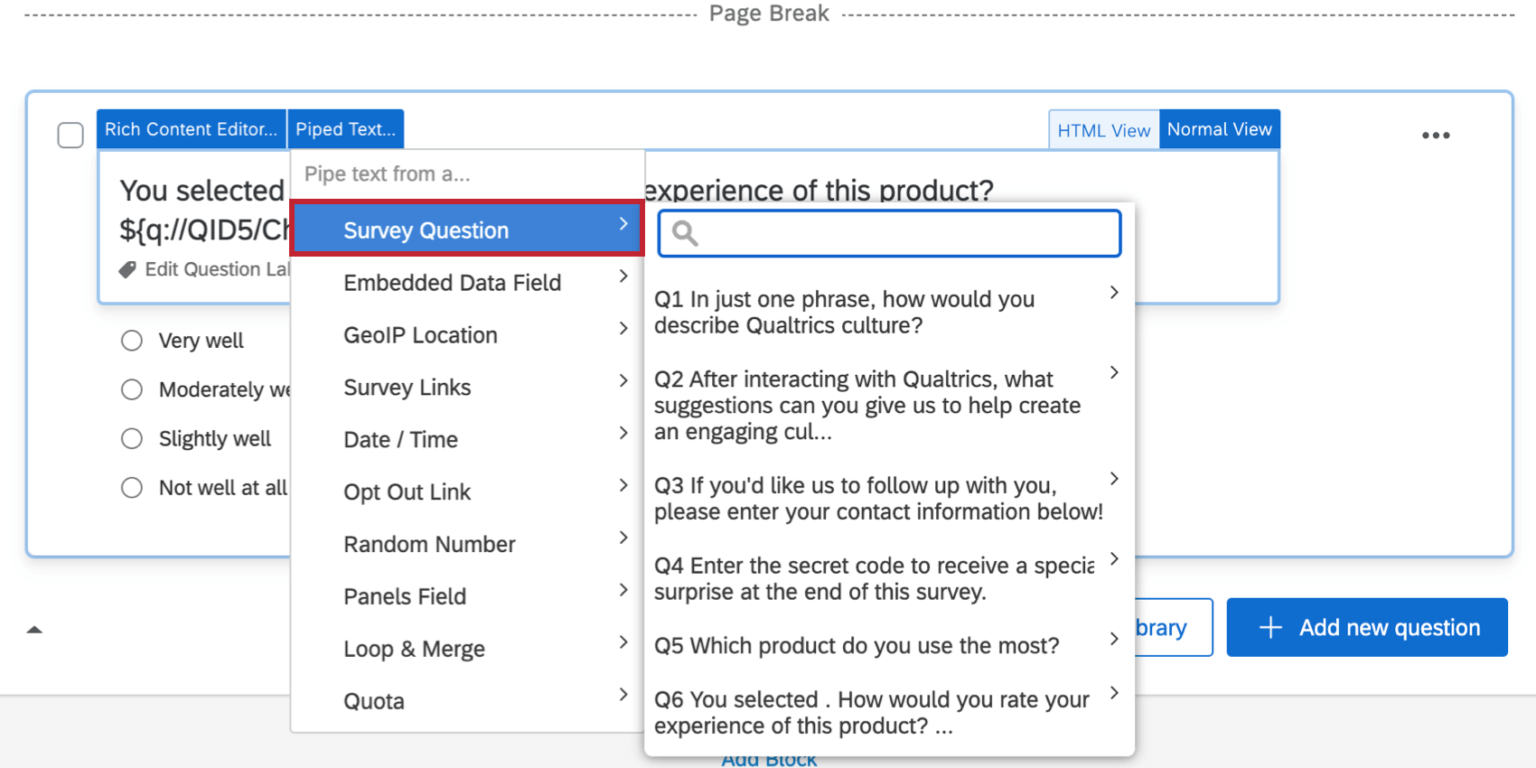A section of a web page is depicted, containing a segment of an online survey editing interface from the Qualtrics platform. In the center of the screen, there's a prominent horizontal divider consisting of a series of dashes with the words "Page Break" embedded in the middle. This element is enclosed in a blue-outlined, white-background box that highlights its function as a page separator within the survey editor.

Above this separator, the interface shows various editing tools. On the left, two blue buttons with white text are labeled "Rich Content Editor" and "Piped Text." Adjacent to these are buttons labeled "HTML View" with a white outline and blue text, and "Normal View" with a blue background and white text, indicating different editing modes available to the user. On the far right of this toolbar is a context menu represented by three vertical dots, suggesting additional options are available.

In the background, a section titled "Cache Queue" with partial visibility indicates that the user is working within a queue, labeled with an ID that is partially cut off. 

Below the separator, the survey builder interface is elaborately detailed. The "Piped Text" option is currently selected, allowing for dynamic text insertion within the survey. Various data fields such as survey questions, embedded data fields, and attributes like IP location, survey link, state, time, and opt-out links are presented as options. These options enable a detailed level of customization for the survey.

To the right, there's a survey question highlighted with a blue background and white text, underlined in red, emphasizing a high-priority or selected item. The question asks, "In just one phrase, would you describe the Qualtrics culture after entering Qualtrics?" suggesting an open-ended response field aimed at capturing qualitative data about user experience.

At the bottom right corner of the interface lies a blue button with white text and a plus sign, labeled "Add New Question," allowing users to seamlessly incorporate additional survey items.

Lastly, on the bottom left, there are multiple-choice responses available, likely for a different survey question, with options ranging from "Very Well" to "Not Well At All." These answer choices have yet to be selected, indicating they are part of an ongoing survey creation process.